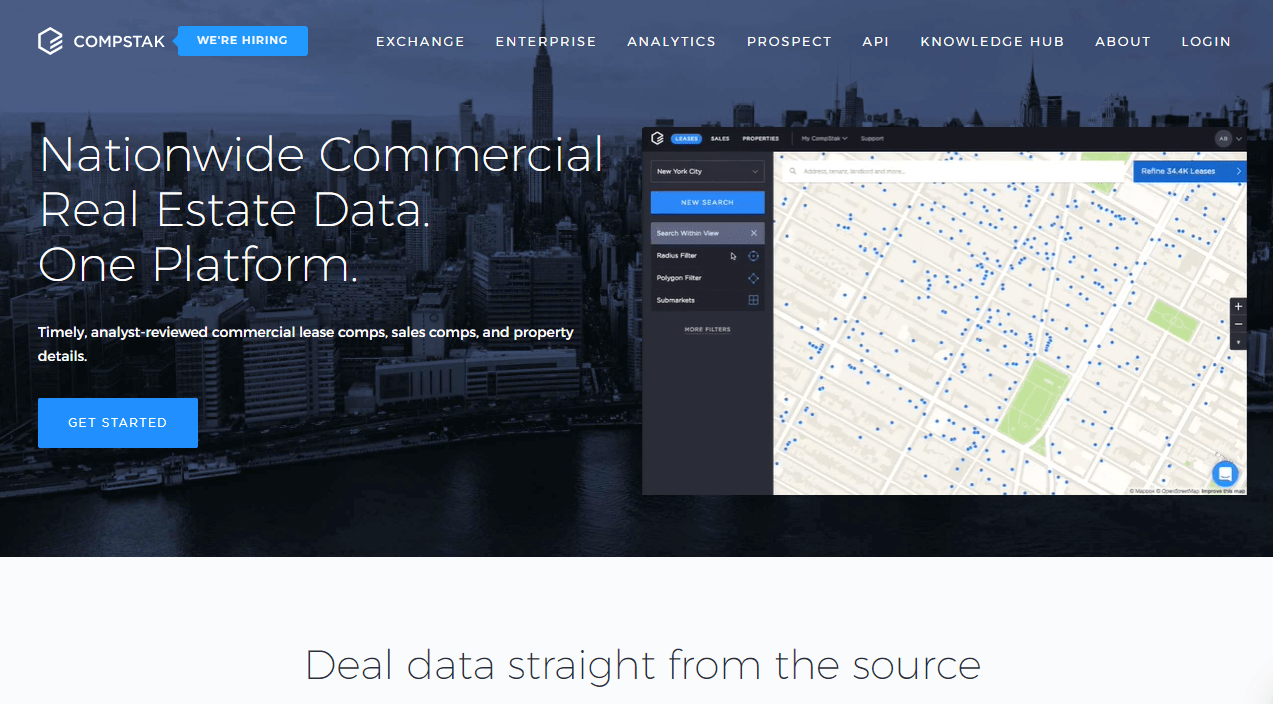The screenshot captures a computer screen displaying a webpage, likely related to commercial real estate data services. At the very top is a large header with a blue background depicting a cityscape, featuring numerous buildings with one particularly tall structure dominating the center. In the upper left corner, the text "CompStak" is visible alongside a blue button labeled "We are hiring." 

To the right, an array of menu options is displayed, including "Exchange," "Enterprise," "Analytics," "Prospect," "API," "Knowledge Hub," "About," and "Log In." On the left side of the image, large text reads "Nationwide Commercial Real Estate Data, One Platform." Beneath this, smaller text lists features such as "Timely," "Analyst Reviewed," "Commercial Lease Comps," "Sales Comps," and "Property Details." A blue button below this text invites users to "Get Started."

The right side of the image features a tan-colored map dotted with numerous blue markers, interspersed with a few green rectangles. At the very bottom, a white background hosts the slogan, "Deal Data Straight from the Source." Returning to the map, to its right, a blue-highlighted button labeled "New Search" suggests an active or selected state, indicating that a user has recently interacted with it.